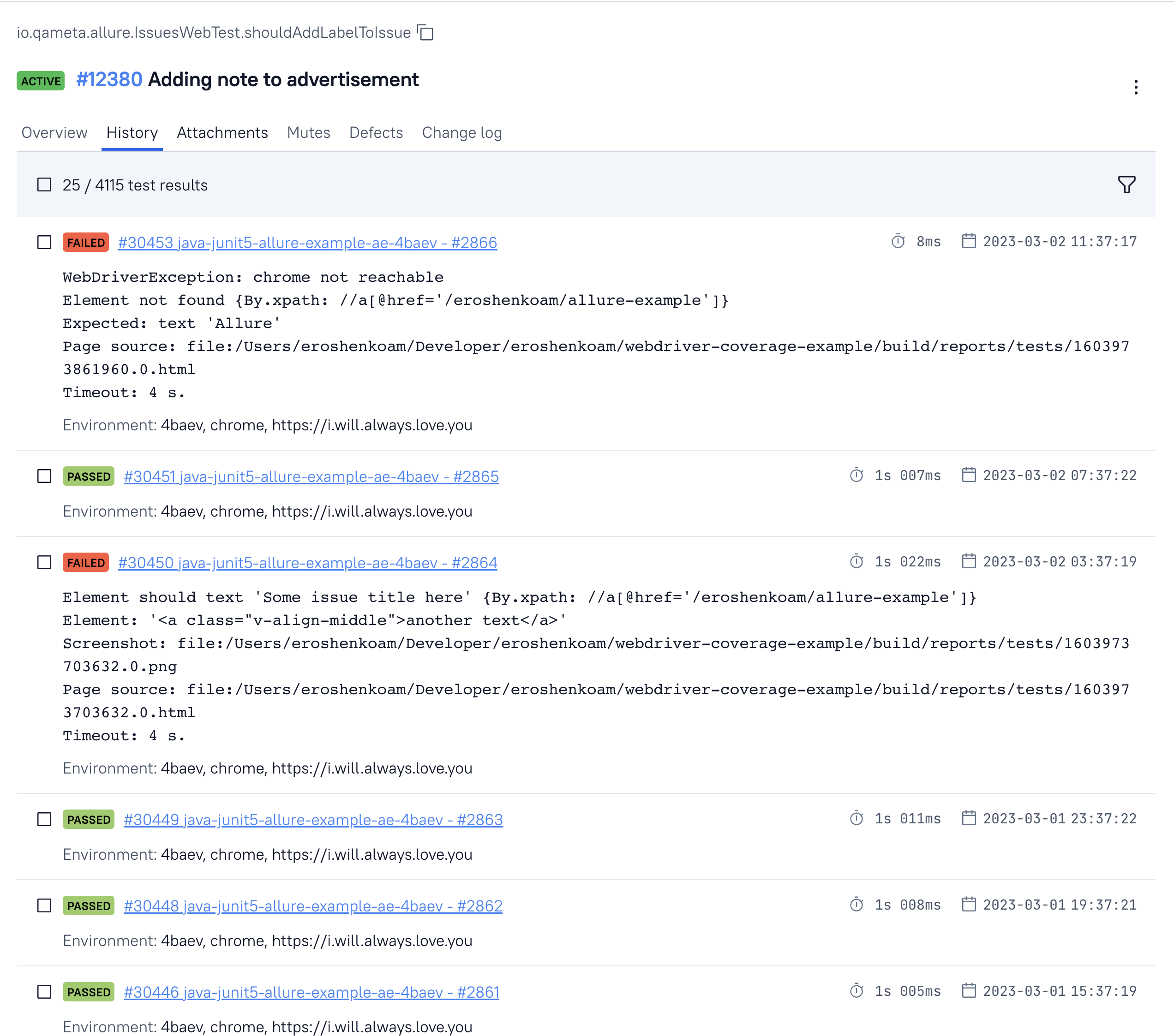A detailed log of a developer's activity is displayed on a laptop or computer screen. The browser tab is labeled "io.quameta.alera.issueswebtest.shouldaddlabeltoissue." At the top right corner, a green-highlighted marker labeled "Active" is visible, followed by the issue number "#12380" and a note titled "Adding note to advertisement." Below this, a navigation bar offers several options: "Overview," "History," "Attachments," "Mutes," "Defects," and "Changelog," with the "History" tab currently selected and underlined in blue. The contents of the screen provide a detailed log indicating a "failed Java on 2023.3.2" entry, suggesting an error or problem encountered during that date. The log appears to contain extensive coding details, including file paths like "file/users/developer," hinting at developer activity and troubleshooting records.